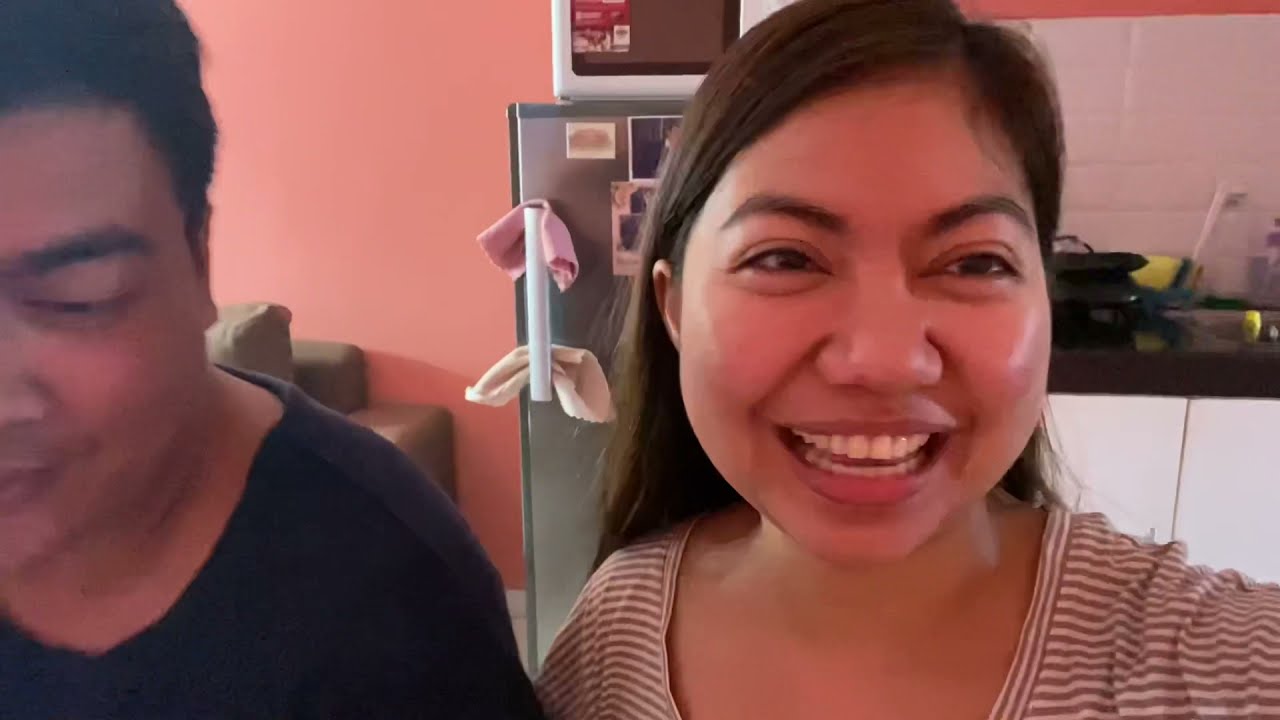A close-up photo captures a smiling woman and a partially visible man, seemingly in a kitchen. The man is on the left side with only the right half of his face showing; his eye is closed, revealing a thick bushy black eyebrow, and he has longish flat black hair. He's wearing a dark shirt. The woman, positioned to the right and in the center of the frame, showcases her shoulder-length or slightly longer dark brown hair and a vibrant smile that reveals both her teeth. She has soft curvy eyebrows and wears a white and gray striped shirt with a v-neck. 

Behind them, a black, stainless steel refrigerator is visible, featuring a white handle with a cloth draped over it. On the top half of the fridge, several white stickers and two photos are prominently displayed. A white microwave rests above the refrigerator, partially obscured by the stickers. To the right, the kitchen continues with white cabinets featuring black tops, and there appears to be a dish or item resting against the cabinet’s edge. Further in the background, a door is visible, indicating another room with peach-colored walls. The lively scene suggests they might be a couple taking a selfie amid their cozy kitchen setting.